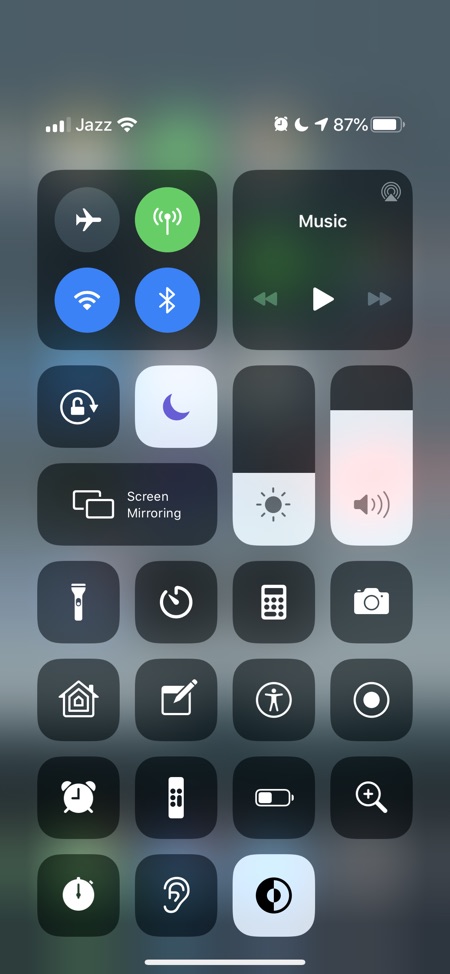This image captures a detailed view of a smartphone's settings menu, displayed upon swiping down from the top of the screen. The background is slightly blurry and predominantly black, with subtle illumination peeking through beneath. 

In the top-left corner of the screen, the word "Jazz" is visible in white font, flanked by various icons on either side. On the upper-right, the battery status reads 87%, displayed both numerically and as a nearly-full white battery icon.

The settings menu is organized into various sections. At the topmost, there's a vertical rectangular area containing four circular icons. The first icon, an airplane within a black circle, likely represents Airplane Mode. Adjacent to it is a green circle icon, followed by two bright blue circles below. The first blue circle features three diminishing lines in a Wi-Fi-like symbol, and the second blue circle's icon is unclear.

To the right of this section is an identically sized square labeled "Music" in white lettering. This area includes a play button shaped like a right-pointing triangle, along with left and right-pointing arrows—likely song navigation controls.

Continuing to the next row on the left side, there is a black circular button depicting a lock with a surrounding arrow pointing downwards—potentially a screen lock button. Adjacent to it is a white button with a purple moon icon, which might represent a Do Not Disturb mode. Below these, a black horizontal rectangle labeled "Screen Mirroring" in white font shows an icon of two rectangular screens with white borders and black centers.

Further down on the left, there are several black circular buttons featuring distinct white icons: a flashlight, a clock, a house, a notepad with a pencil, another alarm clock, and an ear icon.

Beneath the original "Music" square, two vertically aligned rectangular buttons appear. The first button, partially white from the bottom to nearly the midpoint with a sun icon, likely adjusts brightness levels. The second button, almost entirely white with a megaphone-like icon, controls the volume.

Towards the bottom of the settings menu, more black circular buttons are visible: a calculator, a camera, a person inside a circle, a large white dot within a circle, a battery symbol, and a magnifying glass with a plus sign. Additionally, on the left side, a white button features an unclear black and white icon inside it.